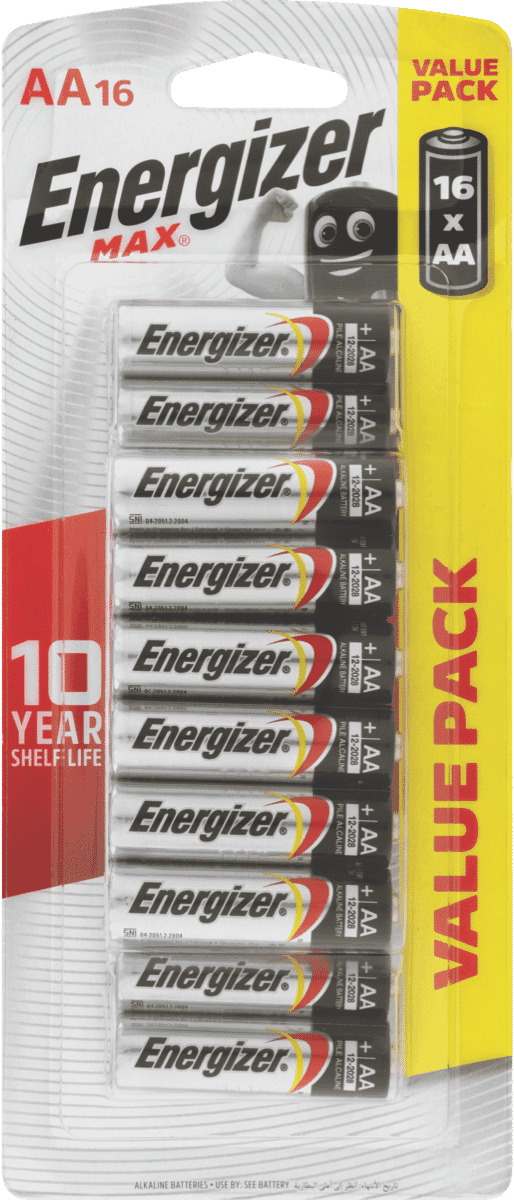The image depicts a package of Energizer Max AA batteries. The packaging features a color scheme of red, yellow, and a light metallic silver-gray. The rectangular package has a rounded top with a hole designed for hanging on retail hooks. The package prominently displays "AA-16" on the side and "Value Pack" in red text at the top right corner, with the term repeated both horizontally and vertically. 

At the center, there are ten AA batteries arranged vertically in clear plastic packaging. A black battery icon with the text "16 x AA" sits above them. A red banner on the left side highlights a "10-year shelf life." Adjacent to this banner is a whimsical illustration of a black battery with a smiley face, flexing a muscular white arm. The background of the packaging is white with a subtle radial line pattern. The overall backdrop of the image is also plain white, making the package details stand out clearly.